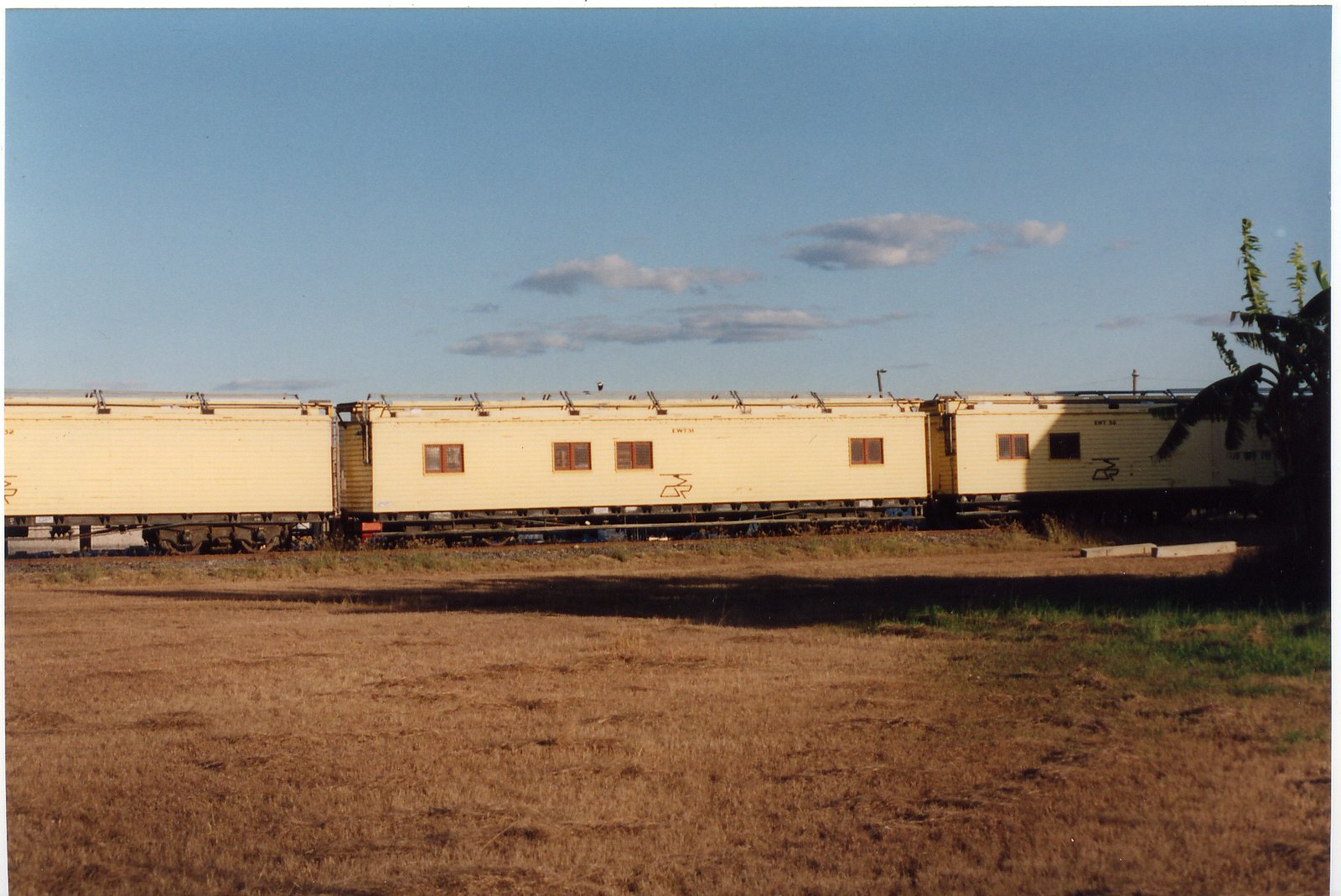This image captures a three-car train in an outdoor setting on a sunny day. The tan or ivory-colored train cars, each adorned with colorful graffiti, feature windows with red moldings separating them. The train is shown on wooden railroad track ties, and it is unclear if the train is in motion. Surrounding the train is a primarily dirt landscape with patches of dried, brown grass and a small area of fresh grass. On the right side of the image, a bush or tree casts a shadow onto the ground. The sky above is a clear blue with a few puffy clouds, creating a bright and well-lit scene.